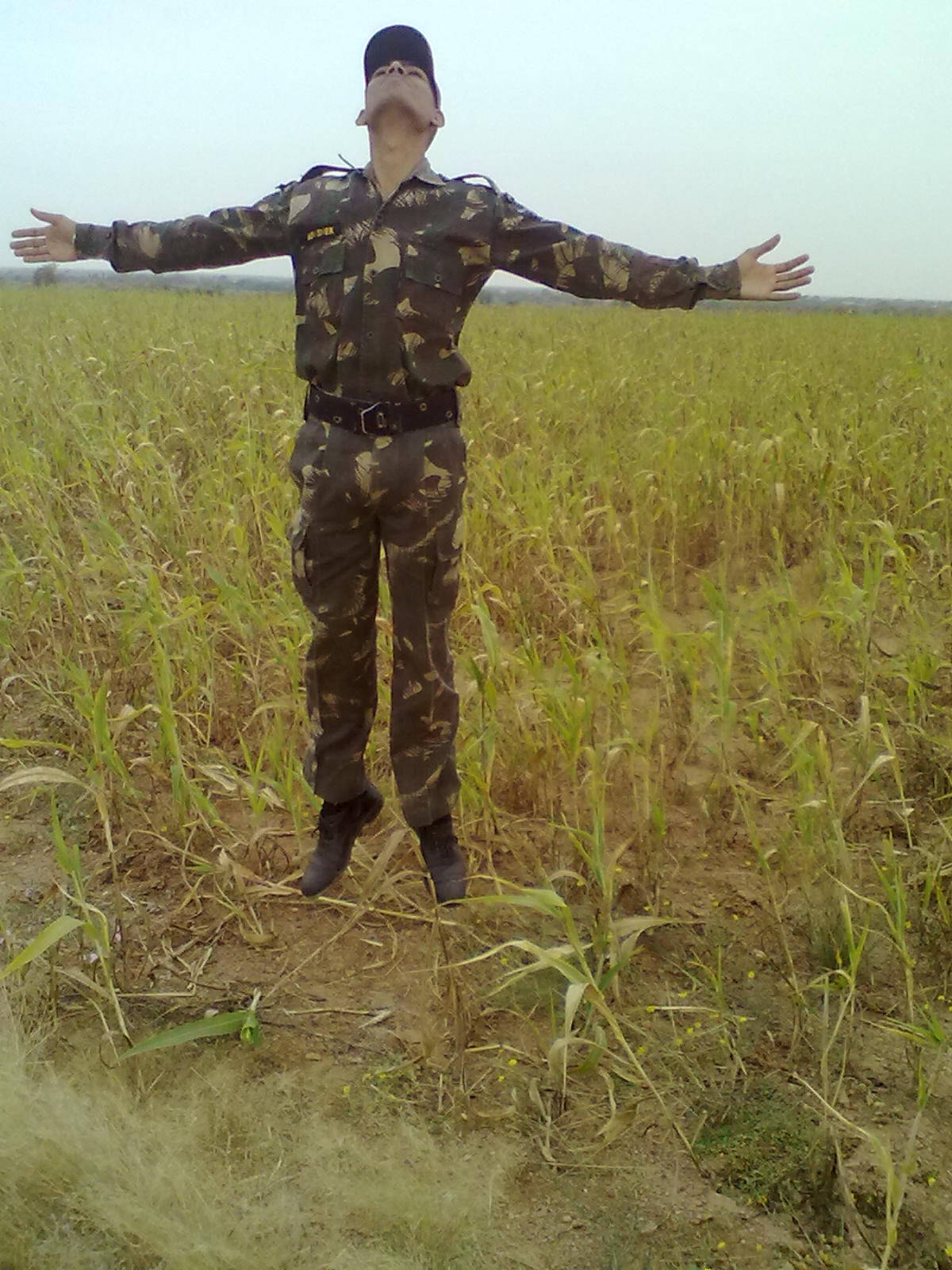The photograph depicts a soldier standing in a field of overgrown grassy vegetation, with his arms extended outwards and his hands held up. He appears to be looking upwards towards a clear, light blue sky, giving the impression of prayer or perhaps a moment of contemplation. His military uniform is a combination of olive and beige camouflage, accentuated with a black belt and black boots. The soldier, with tan-colored skin, which is not pale but distinctly not black, wears a dark green cap that shadows his lifted face. His posture on his tiptoes gives a surreal appearance as if he's slightly levitating. Despite the detailed camouflage and visible name patch on his chest, his face remains obscured, adding a layer of mystery to his identity. The scene is an open, grassy area that is seemingly serene and devoid of additional elements, focusing entirely on the soldier's poignant stance.